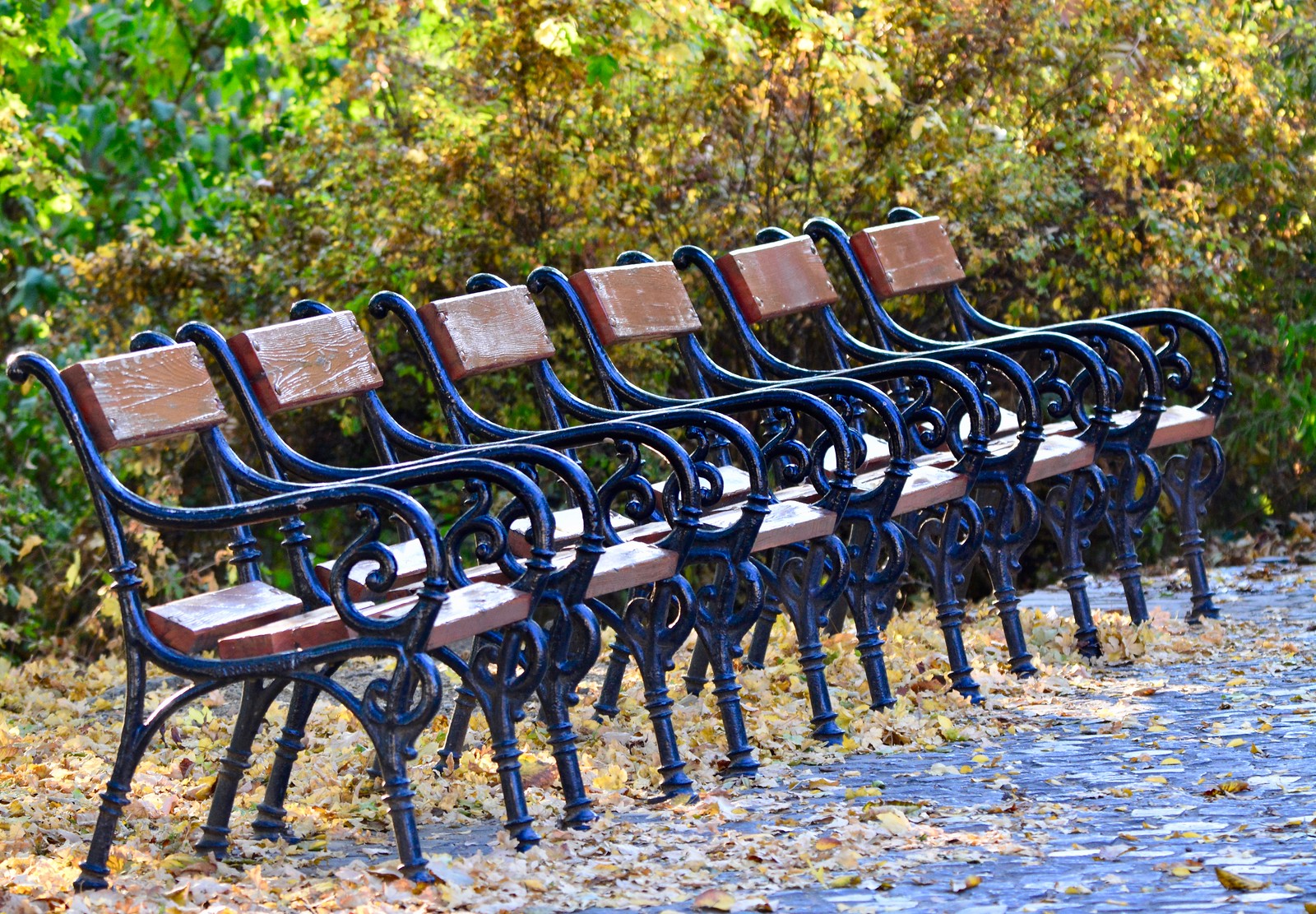The photograph captures a row of six distinctive park benches, arranged diagonally from the bottom left corner towards the top right, though not quite reaching it. Each bench is crafted from wrought iron with ornate, curly cues and detailed arms and legs, lending a touch of antiquity. The seats and backrests are composed of dark brown wood, slightly weathered and fastened securely to the metal frames. The ground beneath the benches is strewn with fallen, golden-brown leaves and patches of dead grass, interspersed with blackish dirt and cobblestones. The background features a lush array of vegetation in autumn hues, including varying shades of green, yellow, and brown, with some sections of plants and bushes showing signs of drying out. This vibrant scene suggests the benches are positioned in a park, set against the rich tapestry of seasonal foliage.